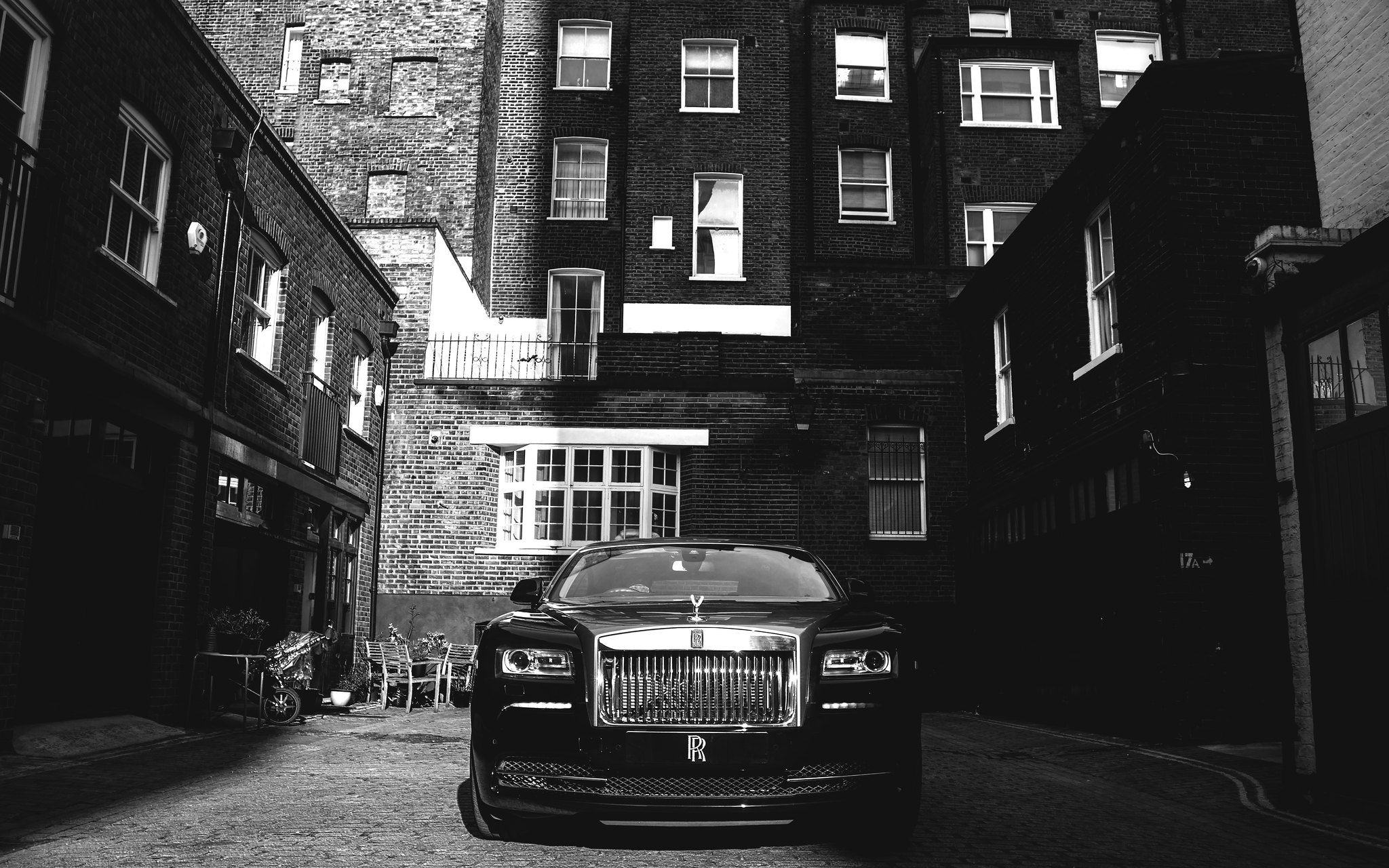In this striking black and white photograph, a Rolls-Royce takes center stage, its sleek black body and iconic chrome front grille immediately drawing the viewer's attention. The car is parked on a brick street resembling a wide alley, positioned in front of an architectural mix of buildings. To the right, a towering dark building with numerous windows lends a shadowy contrast, while a lighter gray building with fewer windows stands to its left. Further left, a shorter, darker structure, potentially a shop or garage, completes the urban landscape. The photo balances light and shadow, with the right side shrouded in darkness and the left illuminated, highlighting the meticulous details of the car and the surrounding structures. Subtle elements such as a wall-mounted camera and a hand truck’s wheel can be detected upon closer inspection, hinting at a deeper narrative within this urban scene.